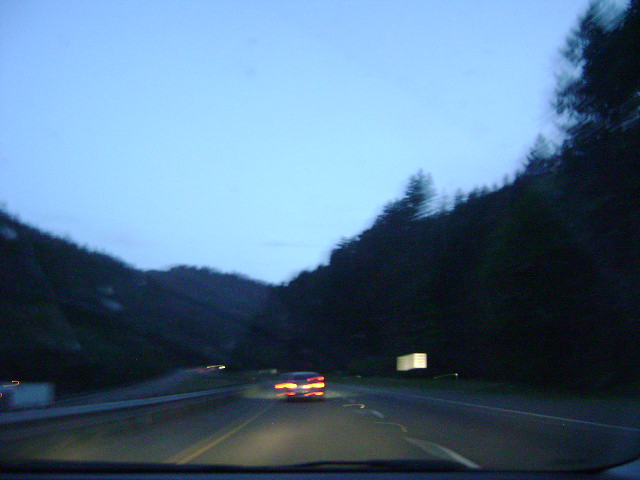The image depicts a scenic highway, possibly captured during early morning or late evening. The sky is tinged with a soft light, suggesting either dawn or dusk. The road cuts through a mountainous region, flanked by lush greenery and tall trees. The photo is slightly blurry, but it shows a car ahead with its headlights and taillights illuminated. To the left, the dark silhouette of the mountains rises, covered in dense, green foliage, while on the right, tall trees and green shrubs dominate the landscape. A highway sign is visible among the trees on the right. The left side of the road features the opposing lane separated by a guardrail, ensuring safety from oncoming traffic.